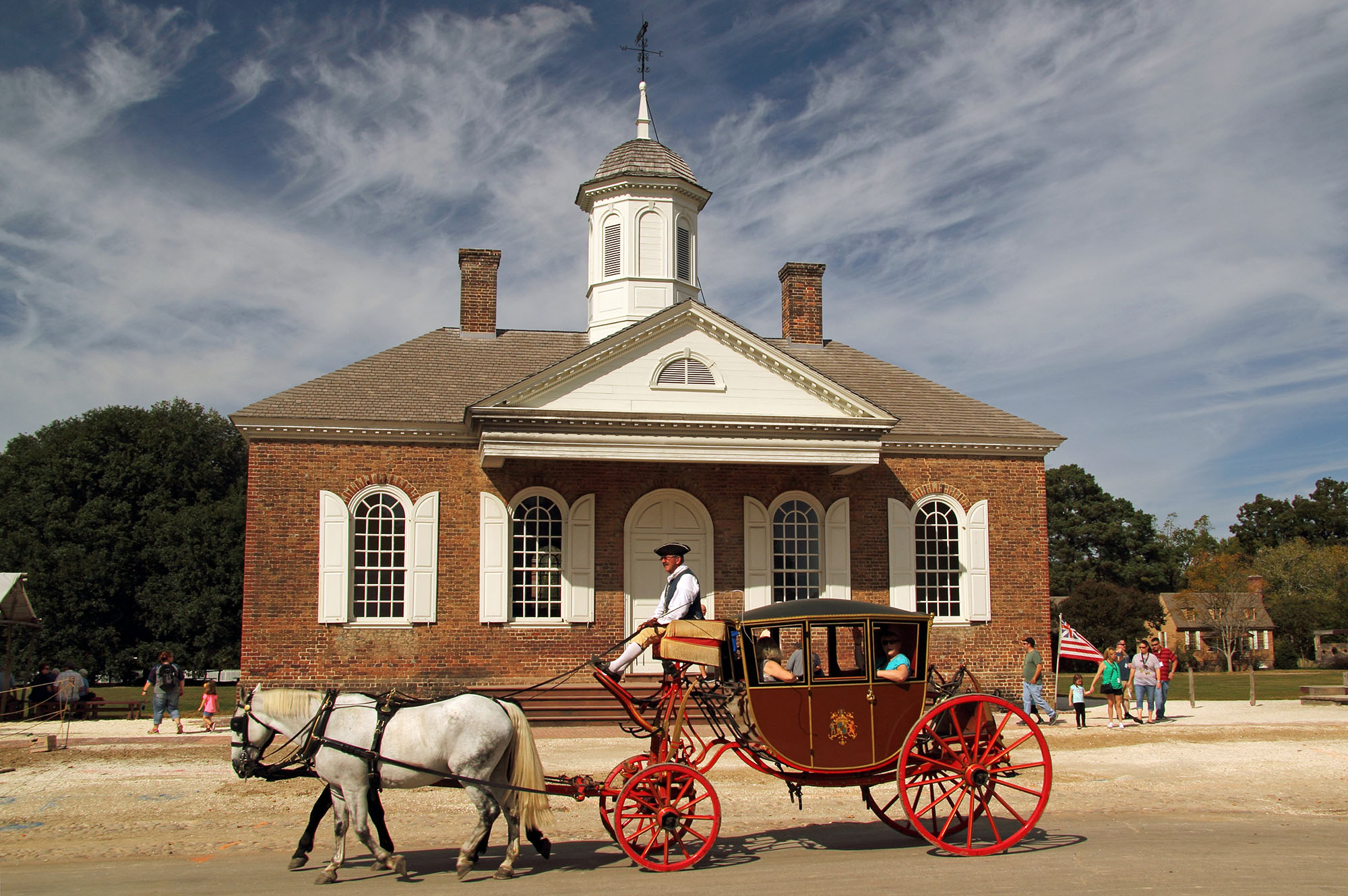The photograph features a historical building showcasing ancient architecture with a prominent sloping roof and a striking tower capped by a grayish-brown dome. At the peak of the structure is a notable spire. The building presents a temple front with four arched, white-painted windows flanking an arched central door, all set against red brick-like walls. The brown-colored sloping roof adds to the visual appeal.

In front of the building, a Victorian-style horse carriage, painted red, is being drawn by two horses—a white horse on the left and a darker horse on the right. The horse guard driver, dressed in black and white period attire and wearing a hat, guides the carriage which carries tourists. The carriage features four wheels, with the front wheels smaller than the rear wagon wheels.

The scene is bustling with people dressed in modern clothing, milling around the building and the flagpole displaying the British flag to the right. In the background, trees add to the picturesque setting. The sky above is a vivid blue, dotted with numerous white clouds, completing the vibrant outdoor scene, marked by a dirt road in the lower third of the photograph. This keenly juxtaposes the timeless charm of historical architecture with the lively movement of contemporary visitors.